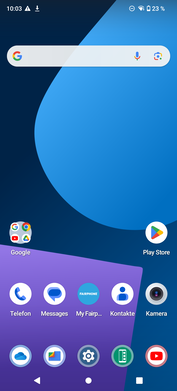A detailed screenshot of a smartphone home screen captured at 10:03 AM. At the top left corner, the time "10:03" is displayed next to a small triangle icon. The top right corner features standard phone status icons: Wi-Fi signal, battery percentage at 23%, and additional network indicators.

Beneath these status symbols lies a large, horizontally elongated Google search bar. This bar is predominantly whitish-gray, with a multicolored "G" logo on its left and a microphone icon paired with a colorful square bearing a circular arrow icon on its right.

The background is a gradient of blue hues, with the left side displaying a deeper blue that transitions to a lighter blue towards the upper right, resembling a large, water-droplet shape. Additionally, in the bottom left corner, a small purple, somewhat square-shaped section is visible.

At the very bottom of the screen, several app icons are lined up in a row. On the left side of this row, a dark blue icon with multiple Google symbols below the text "Google" is situated. Next to it is a white circle featuring the Play Store icon – a multicolored triangle – and the label "Play Store."

Below the primary row of apps is a secondary row featuring circular icons: a telephone icon labeled "Telephone," a message bubble icon labeled "Messages," a camera icon, YouTube icon, and additional app icons including a cloud symbol.